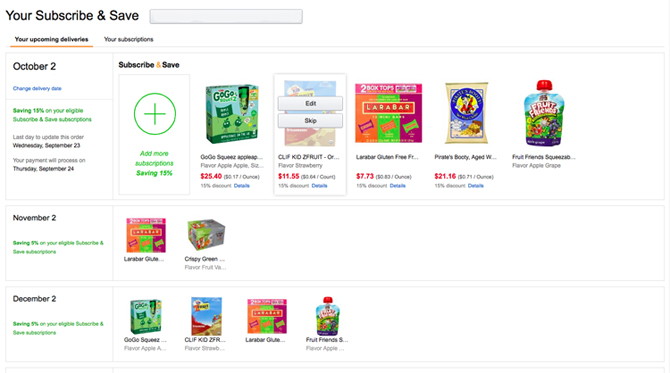The image is a screenshot from Amazon illustrating a person's "Subscribe & Save" page. At the top left, in black text, it states "Your Subscribe & Save." Directly below, the heading "Your Upcoming Deliveries" is displayed, followed by "Your Subscriptions." The person has selected the tab for "Your Upcoming Deliveries."

For the delivery scheduled on October 2nd, the page shows several important details. In black text, the delivery date is mentioned as "October 2nd." In blue text, there is an option to "Change Delivery Date," while in green text, it indicates a saving of 19% on eligible "Subscribe & Save" subscriptions. Additional information includes the last day to make updates and when the payment will be processed.

The product list for October 2nd includes a $25 pack of GoGurt, which the person has clicked on, allowing them to either edit or skip the item. Other products scheduled for this delivery include Lara Bars, Pirate's Booty Popcorn, and fruit squeezes.

For the upcoming delivery on November 2nd, the list includes more Lara Bars and a product named Crispy Green, although the exact type of Crispy Green product is unclear.

Finally, the December 2nd delivery includes more Clif Bars, fruit squeezes, and a few other unspecified items.